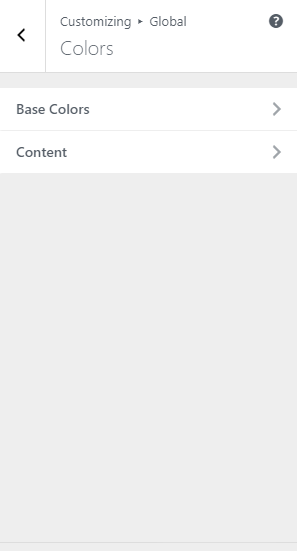The image depicts a user interface, likely from a web page or an application, characterized by its minimalistic and predominantly gray and white color scheme. At the top of the screen, the heading "Customizing Global" is prominently displayed, with an arrow pointing to the word "Global." In the upper right corner, there is a circular icon featuring a question mark, indicative of a help or information feature.

Just below the main heading, the word "Colors" is displayed, followed by the label "Base Colors" with an arrow pointing to the right, suggesting that this is a clickable link. Further down, the word "Content" appears, also accompanied by a right-pointing arrow, indicating another link. The lower portion of the screen is occupied by a light gray, rectangular box with no visible content inside.

In summary, the interface includes headings and navigation links for customizing global settings, colors, base colors, and content, with a significant amount of blank space, giving it a sparse and uncluttered appearance.